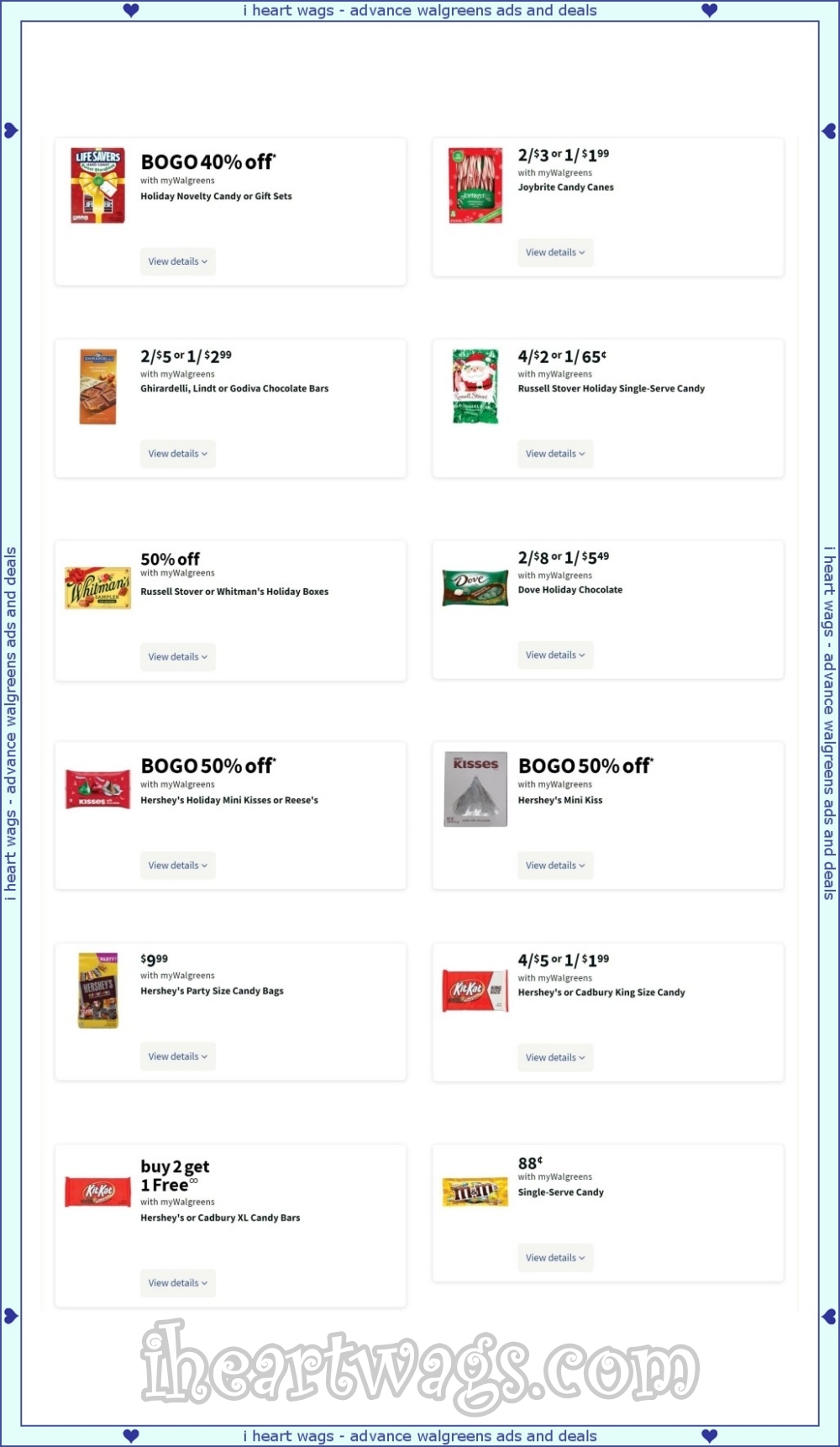**Caption (Under the Category: Websites)**

The webpage features a light blue frame with dark blue trim and small blue hearts scattered throughout. It prominently displays the heading, "iHeartWags," indicating advanced Walgreens ads and deals. 

Highlighted deals include Lifesavers BOGO: Buy one, get one 40% off with MyWalgreens on Holiday Novelty Candy or Gift Sets. A "View Details" link is also provided. Another offer shows Joybrite Candy Canes priced at 2 for $3 or 1 for $1.99 with MyWalgreens, accompanied by an image of a candy cane box. 

Moreover, the site lists deals on premium chocolates: Ghirardelli, Lindt, or Godiva chocolate bars are available at 2 for $5 or 1 for $2.99 with MyWalgreens. There's also a visual of Russell Stover Holiday Single Serve Candy featuring a marshmallow Santa.

Whitman's or Russell Stover Holiday Chocolate Boxes are 50% off with MyWalgreens. Dove Holiday Chocolates are priced at 2 for $8 or 1 for $5.49 with MyWalgreens. 

Additional deals include:
- Buy One Get One 50% off Hershey's Holiday Mini Kisses or Reese's
- Hershey's Party Size Candy Bags at 4 for $5 or 1 for $1.99
- Hershey's or Cadbury King Size Candy Bars
- Hershey's or Cadbury Extra Large Candy Bars for 88 cents 
- Single serve M&Ms with MyWalgreens.